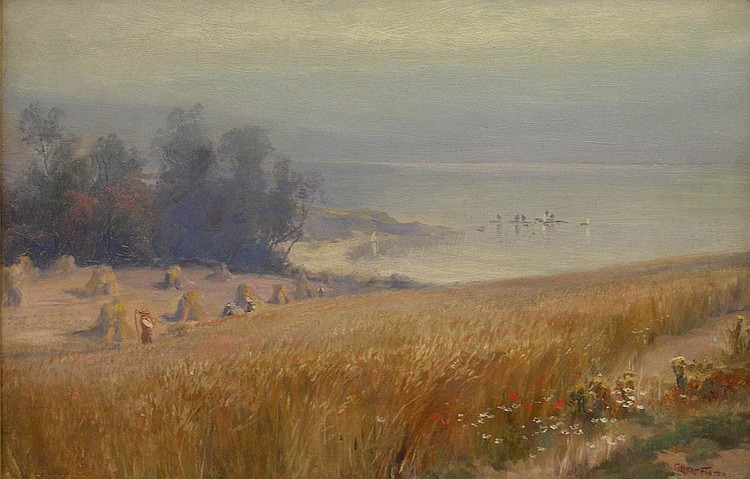This painting, with its vintage and impressionistic style, captures a serene, expansive landscape from a hilltop perspective. The foreground is dominated by tall, brown grasses, likely wheat, interspersed with wildflowers. A farmer, with a scythe over his shoulder, is working the field, and neatly arranged bales of hay are visible at the bottom of the hill. The setting has a warm, autumnal color palette with hues of brown, green, and red, giving the artwork a slightly aged, hazy quality. In the middle distance, there's a lake or ocean, with sailboats and ships anchoring in a harbor area, surrounded by rocky cliffs and edged with a small forest. This serene scene, dotted with trees and small straw huts, evokes a nostalgic, tranquil atmosphere, beautifully blending the elements of nature, agriculture, and coastal life into one harmonious view.